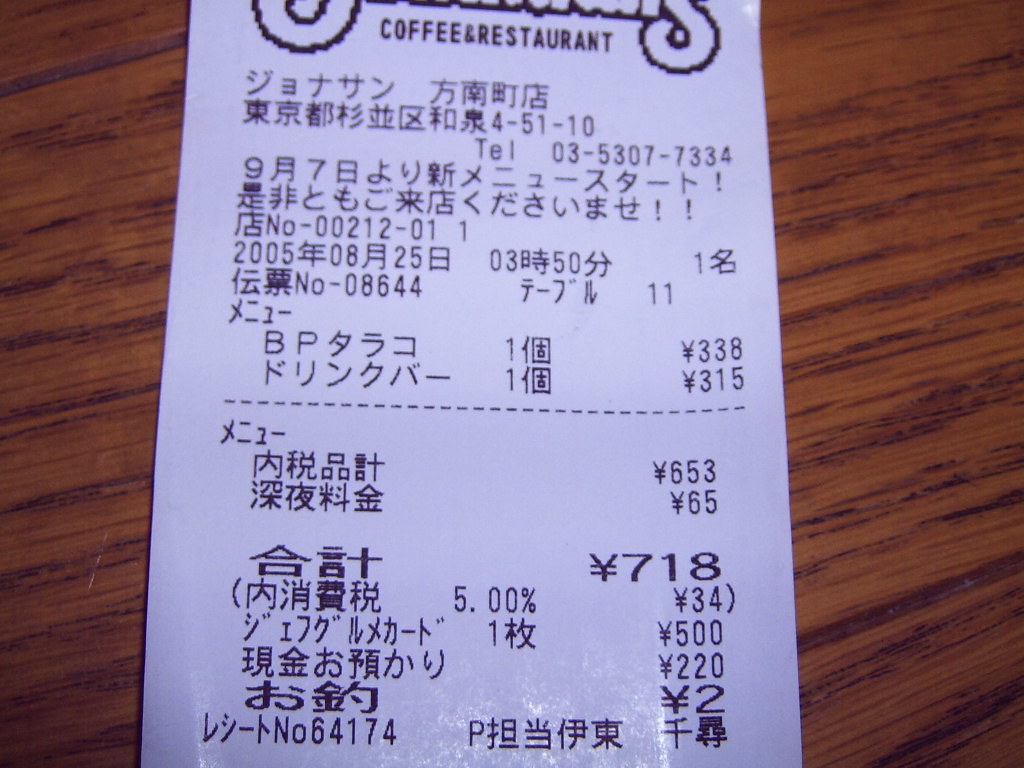A detailed photograph captures a receipt placed on a clean, wooden table. The table features a medium brown shade with darker grooves and lighter sections, emphasizing its wood grain texture. The white receipt, positioned dead center in the image, prominently displays the text "COFFEE AND RESTAURANT" in black, capital letters at the top, though the restaurant's name is not visible. The receipt is predominantly written in Chinese characters, with a few recognizable numbers and details. The left side lists several amounts in yen: 338 yen at the top, followed by 315 yen, and a calculated total of 653 yen. Below this total, an additional charge of 65 yen, likely tax, brings the sum to 718 yen, with a noted 5% charge equating to 34 yen. Additionally, there's a telephone number, 03-5307-7334, visible on the receipt. The very bottom left corner features the number 64174, which might be a store identifier.